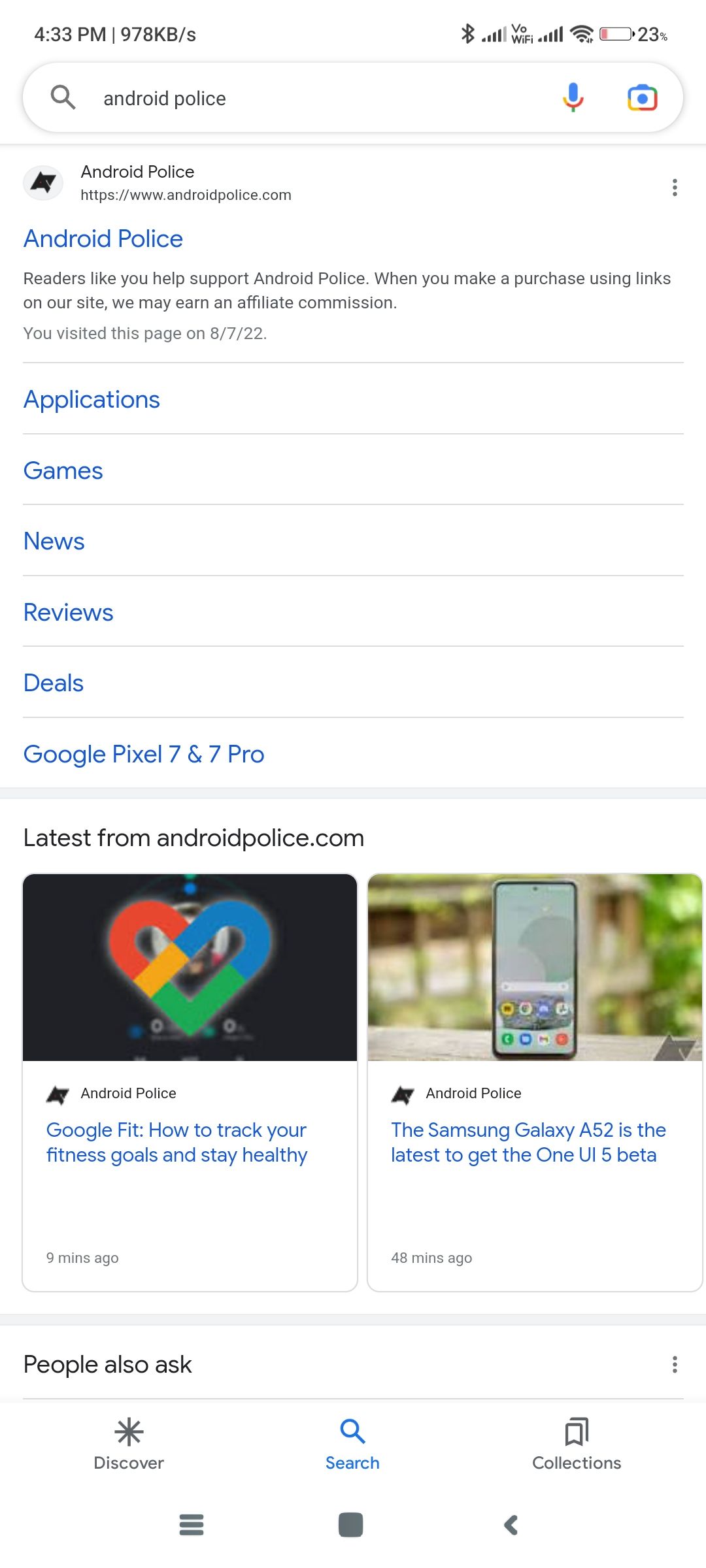This detailed caption describes a screenshot taken from a cell phone displaying various icons, notifications, and content from the Android Police website:

---

The screenshot, taken at 4:33 PM, shows a phone status bar at the top left corner displaying the download speed of 978KB/s. Moving to the right, there are several icons in sequence: a Bluetooth icon, a network coverage icon, a Wi-Fi icon, and a battery icon indicating 23% remaining power.

Beneath the status bar is an oblong search bar. On the left side of the bar is a magnifying glass icon. Inside the bar, the text reads "Android Police." To the right are a microphone icon and a camera icon.

Directly below the search bar, the text "Android Police" appears, followed by the URL "www.androidpolice.com," repeated instances of "Android Police," and a note: "Readers like you help support Android Police. When you make a purchase using links on our site, we may earn an affiliate commission. You visited this page on 8-7-22."

The website's main navigation categories are listed next: Applications, Games, News, Reviews, Deals, Google Pixel 7 and 7 Pro. Following this, the section titled "Latest from androidpolice.com" features two articles:

1. A colorful heart image segmented into red, yellow, blue, and green parts with the label "Android Police." Below the image, the headline reads, "Google Fit: How to track your fitness goals and stay healthy," posted 9 minutes ago.
   
2. An image of a smartphone propped up on a table against an out-of-focus background that seemingly captures trees. Under the image, the text states "Android Police." The headline below reads, "The Samsung Galaxy A52 is the latest to get the One UI 5 Beta," posted 48 minutes ago.

At the bottom of the screenshot, the options "Discover," "Search" (highlighted), and "Collections" are shown under the "People also ask" section.

---

This caption provides a comprehensive and detailed description suitable for someone relying solely on text to understand the content and layout of the captured screen.